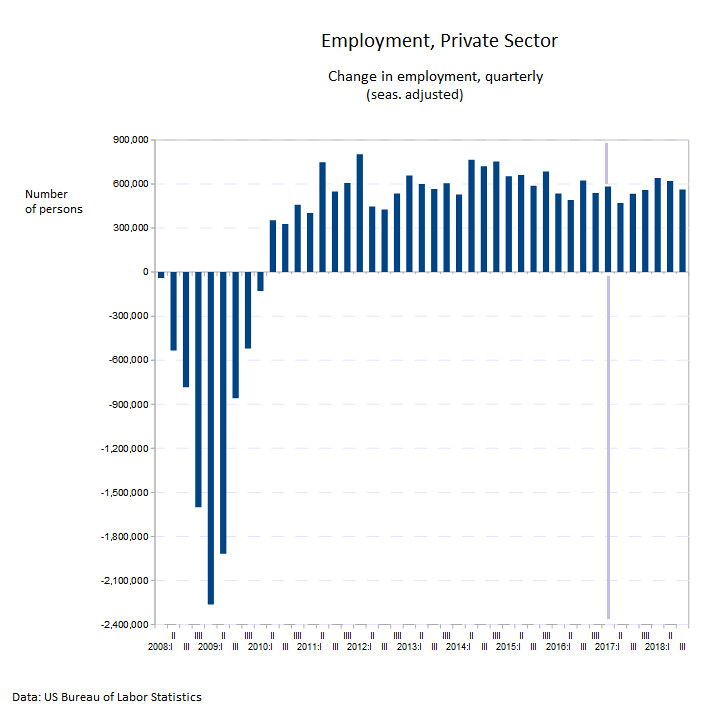The data visualization is a borderless graph on a white or transparent background, featuring a detailed analysis of quarterly changes in private sector employment, seasonally adjusted, from 2008 to 2018. The title of the graph, "Employment, Private Sector: Change in Employment (Quarterly, Seasonally Adjusted)," is printed in black at the top. The y-axis, labeled "Number of Persons," ranges from 900,000 at the top to -2.4 million at the bottom. The x-axis represents time, marked in quarters from 2008 Q1 to 2018 Q3.

The graph displays vertical navy blue bars indicating employment changes, with the bars dipping significantly below zero around 2009, nearly reaching -2.4 million, before gradually climbing back up to zero around 2010. Post-2010, the bars remain above zero, fluctuating between 300,000 and 700,000 for the remainder of the period. A prominent light blue vertical bar appears at 2017, although its specific significance is not noted. At the bottom left corner, the source of the data is cited as the U.S. Bureau of Labor Statistics.